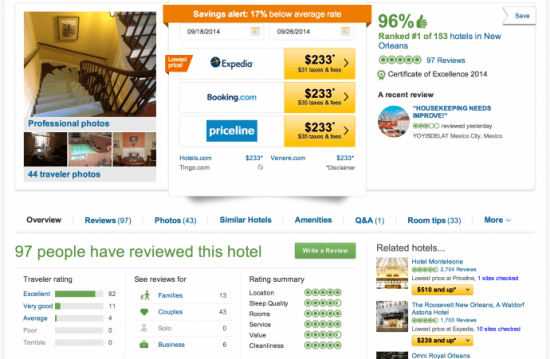**Caption:**
On a bustling webpage dedicated to hotel bookings, a prominent "Savings Alert" banner is displayed at the top center, highlighting that the rates are 17% below average for the dates 9-18-2014 to 9-26-2014. The banner reveals the lowest price available on Expedia at $2.33, plus $31 in taxes and fees, while Booking.com and Priceline offer the same base price with $35 in taxes and fees.

To the left of this central section, a professional photo depicts a long stairway, accompanied by three small thumbnails underneath labeled "3 of 44 traveler photos." This suggests there are 44 traveler photos available in total. 

On the right-hand side of the page, the hotel boasts a high approval with 90% thumbs up and is ranked number one out of 153 hotels in New Orleans. Out of 97 reviews, the hotel averages a five-star rating and has earned a Certificate of Excellence for 2014. A recent less favorable review, however, indicates housekeeping could use improvement, giving only a three-star rating.